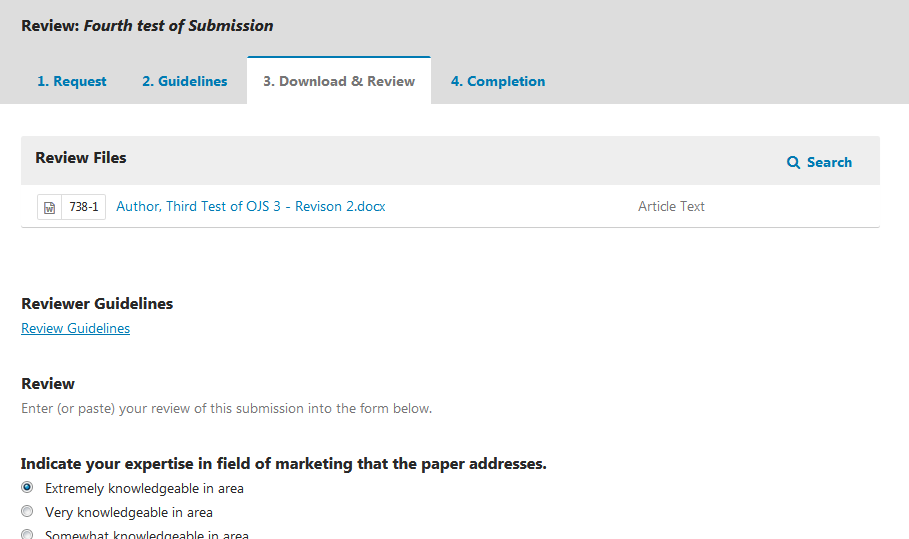Here is a cleaned-up and detailed version of the caption:

"Screenshot of a review interface for a document submission. At the top, there is a gray bar with black text on the left side that reads, 'Review: Fourth test of submission.' Below the gray bar, there are four options displayed as blue links, except for the selected option, which is grayed out and appears slightly raised. The options are: 1. Request, 2. Guidelines, 3. Download and Review (selected), and 4. Completion. 

Beneath these options, users can choose to review files or search for something specific. A document titled 'Author – Third test of OJS 3 revision 2.x article text' is selected for review. Below the document title, there is a section labeled 'Reviewer Guidelines' in black text, with a corresponding blue link titled 'Reviewer Guidelines' underneath it.

Next, in black text, there is a prompt that reads, 'Review: paste your review of this submission into the form below.' Further down, reviewers are prompted to 'indicate your expertise in the field of marketing that the paper addresses.' There are three options provided for this prompt, and the first option, 'Extremely knowledgeable in area,' is chosen."